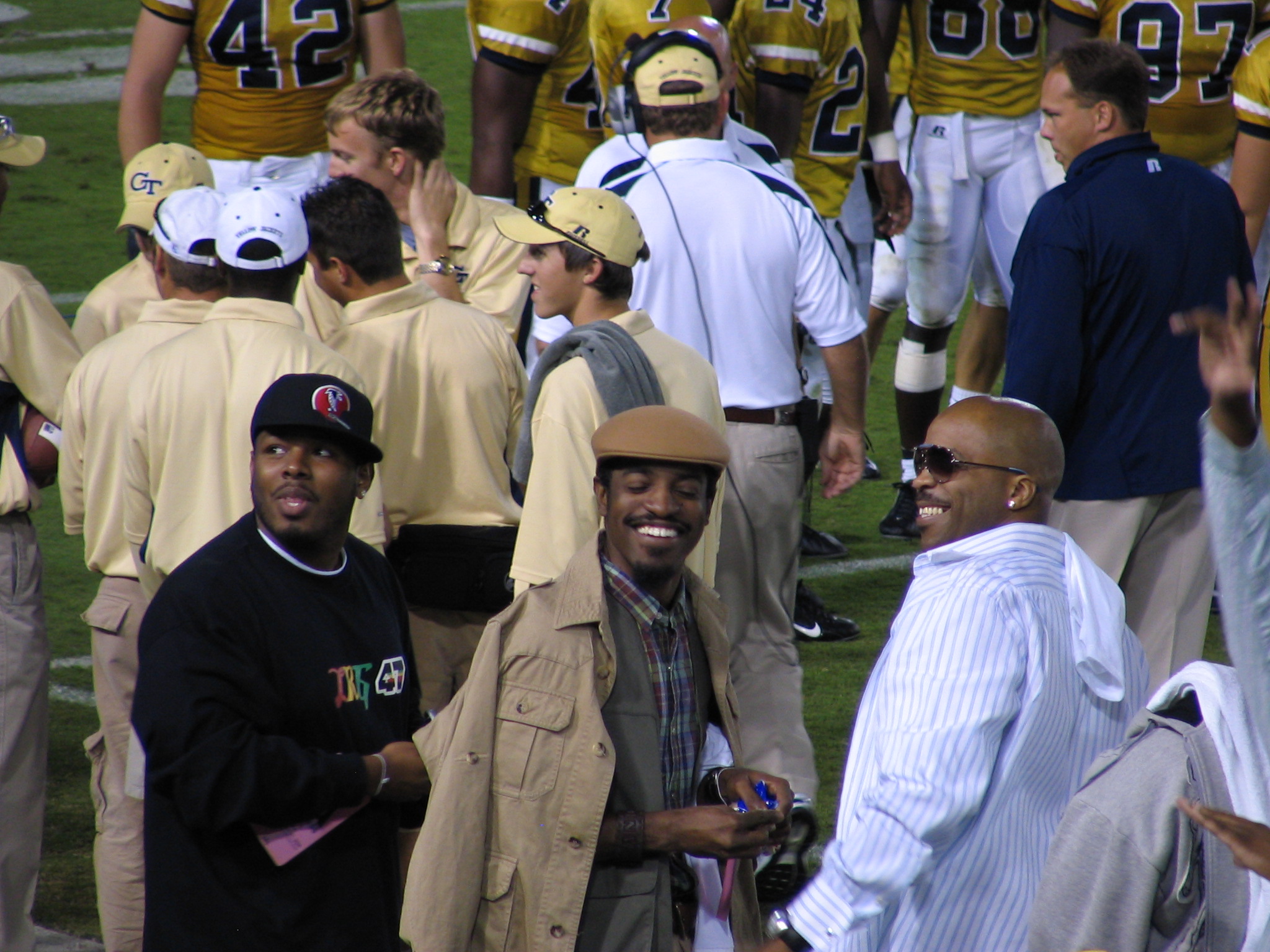In the foreground of the image, three men are the central focus, all smiling and looking back over their shoulders. The man on the left is wearing a long black t-shirt and black hat with a mustache and beard, his open-mouthed smile facing slightly upwards to the left. The middle figure, rapper Andre 3000, has his eyes closed and is wearing a beige beret, a plaid red and blue shirt underneath, and a beige jacket. His wide smile reveals his top teeth, and he holds an unidentified blue item in his hands. The man on the right dons shades, an earring, and a white shirt with blue trim, his smile directed towards the camera. In the background at the top of the image, a football team is visible, with players wearing yellow jerseys and white shorts, out on a green field. Among them, other team members and assistants can be seen moving about, some dressed in white shirts with beige hats and beige polo shirts. The scene captures a lively moment set against the structured lines of the football field.